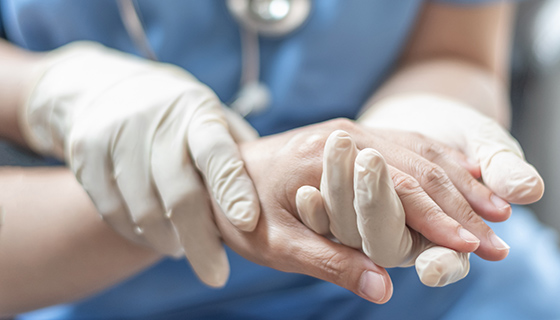In the background of the image, a medical professional is depicted from the neck to the mid-leg, clad in pale blue scrubs with a silver stethoscope draped around their neck. The professional's white gloves, appearing slightly wrinkled and in need of replacement, are gently holding an elderly person's left hand. The elderly hand, also white and visibly wrinkled, rests in the palm of the medical caregiver's left hand. Meanwhile, the caregiver's right hand is tenderly grasping the wrist of the elderly person. This intimate moment seems to capture the act of the medical professional providing comfort and reassurance to the elderly individual, who is likely a patient in a hospital setting.